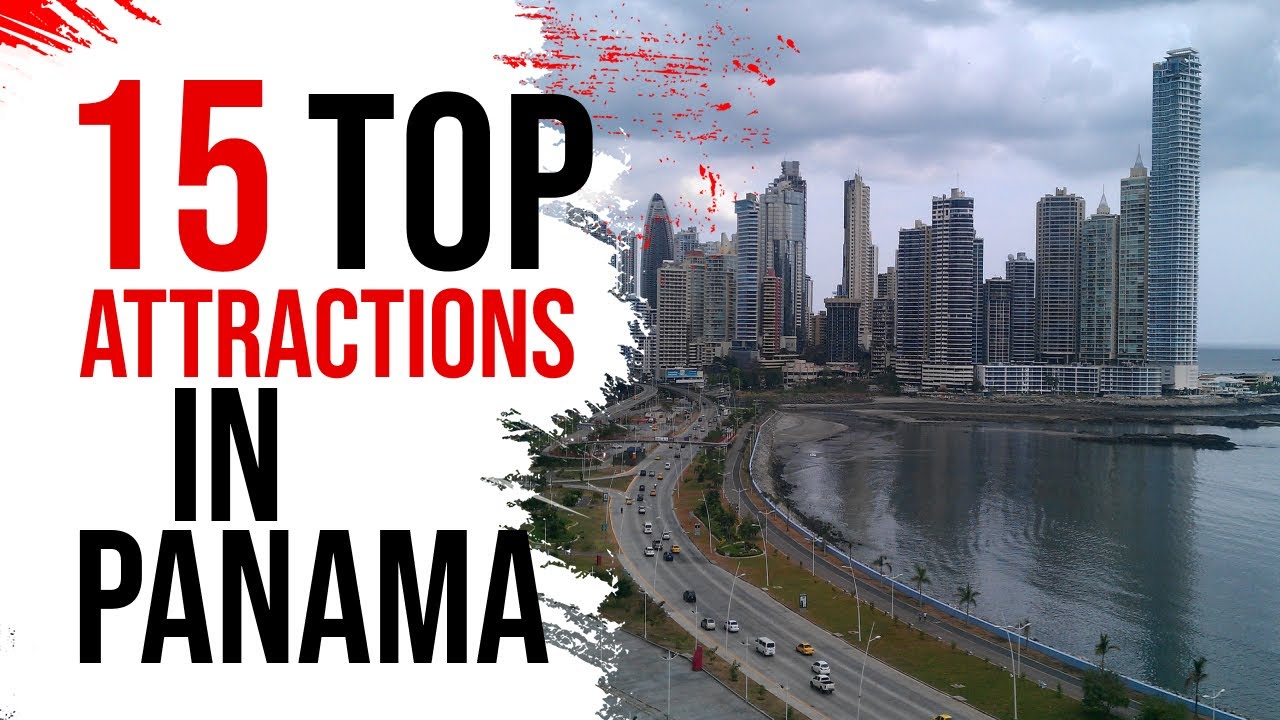The image presents a title header for an article or guide, labeled "15 Top Attractions in Panama." The title features a striking color contrast: the number "15" is in bold red and fully capitalized, while the word "TOP" is in black and also fully capitalized. These two words are placed on the same line. Directly beneath them, the word "ATTRACTIONS" appears in red, fully capitalized, but in a slightly smaller font size. Below this, the word "IN" is displayed in a larger black font and is centrally aligned under the letters "T" and "R" of the word "ATTRACTIONS." Lastly, at the bottom, the word "PANAMA" is written in all black capitals.

The background behind the text is primarily white, allowing the title to stand out. On the right side of the image, there is an artistic touch that transitions into what looks like a partially painted aerial photograph. This photo depicts a bustling urban environment with numerous cars driving out of the city, which is filled with tall buildings and stretches towards the background. The cars are notably positioned towards the bottom of the image, enhancing the impression of movement and dynamism.